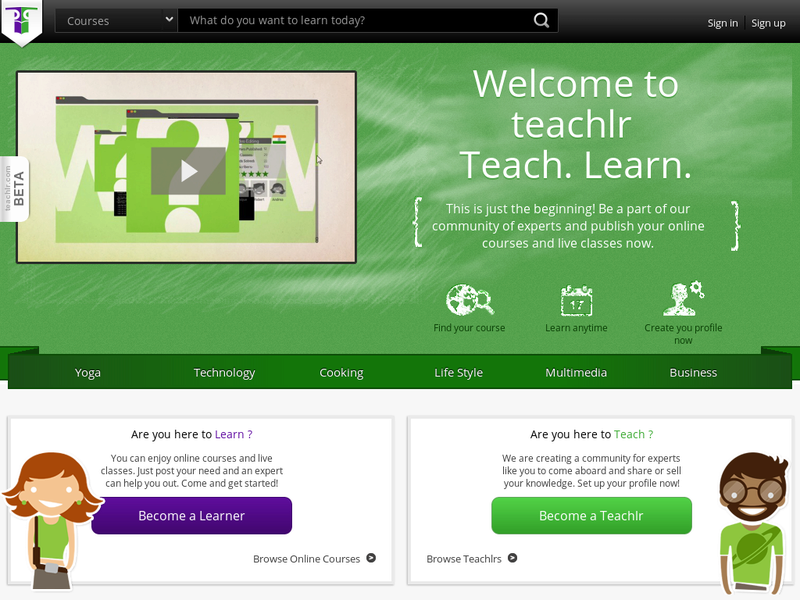The image is a screenshot of the home page of a website called "TeachLR."

The header graphic features a light green, chalk-like texture, adding a fitting theme of education. Prominently on the right side, a white headline reads "Welcome to TeachLR," with "TeachLR" in a lowercase "t" and spelled out as T-E-A-C-H-L-R. Beneath this headline, also in white font, it says, "Teach. Learn." followed by, "This is just the beginning. Be a part of our community of experts, and publish your online courses and live classes now."

On the left side of the header, there is a gray oblong rectangle which appears to be a video player, evidenced by the white play triangle at its center.

Below the header graphic, another darker green bar spans the width of the page, containing a navigation menu with items listed left to right: Yoga, Technology, Cooking, Lifestyle, Multimedia, and Business—all written in white font.

In the lower left-hand corner, set against a white background, a stylized illustration of a woman with red hair in a green tank top is accompanied by the text, "Are You Here to Learn?" Nearby, a purple rectangular button with white text says "Become a Learner."

Conversely, in the lower right-hand corner, another stylized cartoon drawing of a man with brown hair, large round glasses, and a green t-shirt is present. This side features a green button with white text that reads, "Become a Teacher."